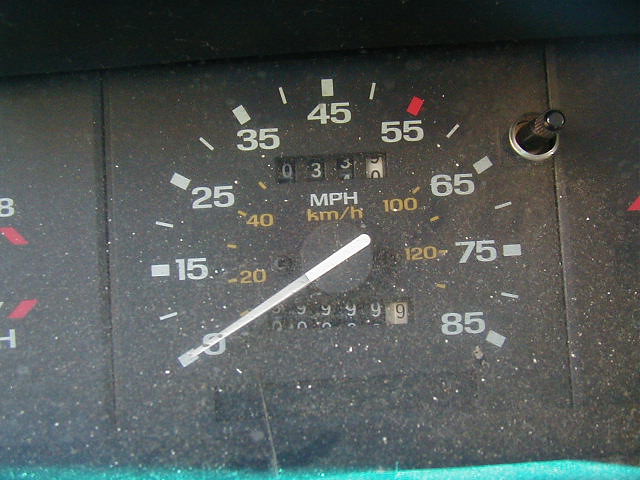This photograph showcases a vintage odometer, believed to be from the 1960s. The odometer is heavily worn, displaying a considerable amount of dirt and rust. The mileage display appears to have reached its maximum limit. The speedometer needle is pointing to 33 miles per hour and is white in color. The odometer numbers are also white, while the kilometer numbers are distinguished in gold. The dashboard, serving as the background, is black. The odometer hand rests at zero. On either side of the speedometer, there are markings: an 'H' on the left and a 'B' on the right, possibly indicating additional indicators or functions. Additionally, a small button or dial is located at the top near the odometer, which might be used for resetting purposes.